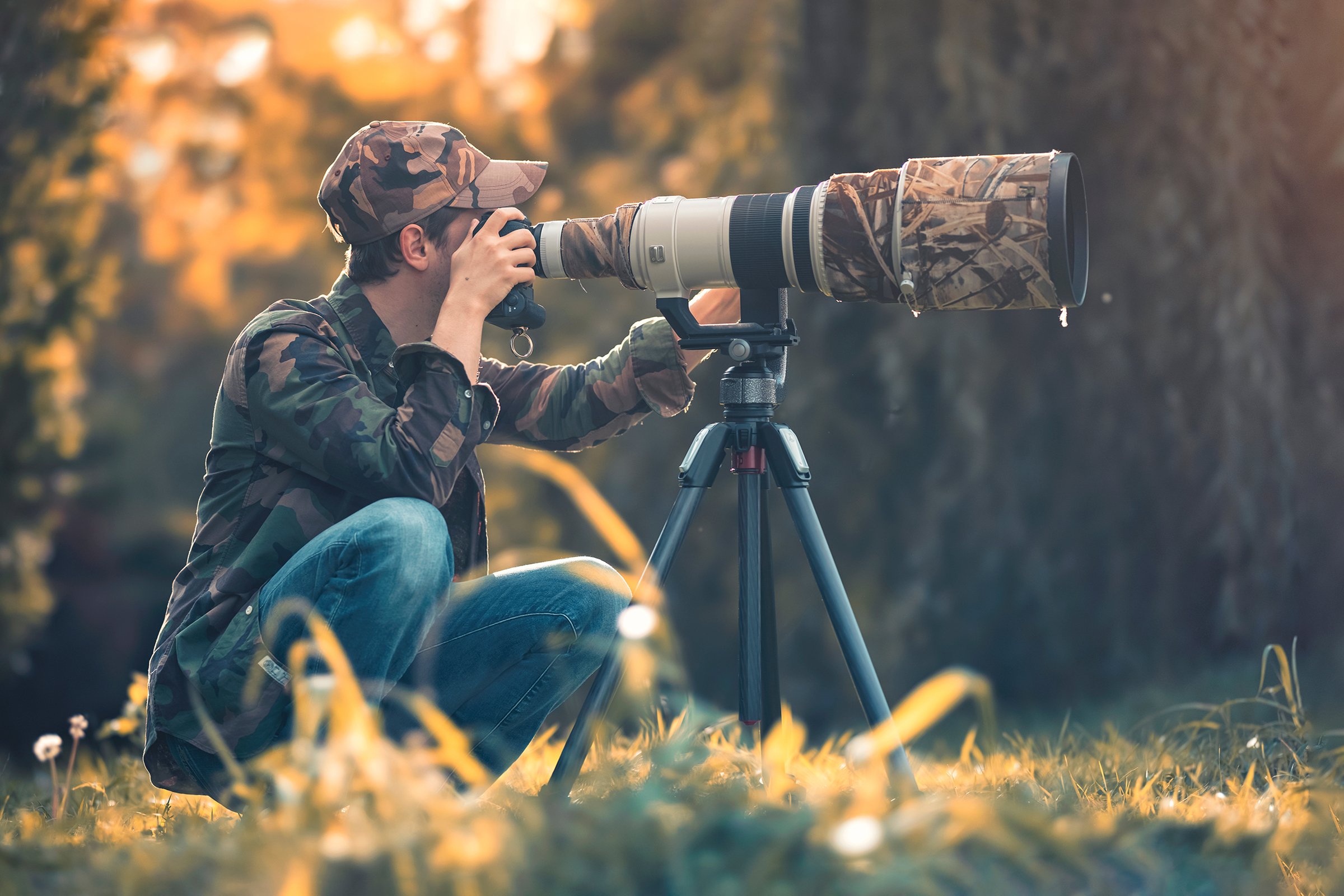The image depicts a man kneeling in the woods, blending into his surroundings with blue jeans and a camouflage shirt and hat that feature shades of green, brown, beige, and black. He is engaged in wildlife photography, using a large, intricate camera setup mounted on a tripod with his right hand on the shutter and left hand adjusting the focus on the telescopic lens. The camera itself has a camouflage pattern with a combination of smooth black, brown, green, and off-white colors to match the natural environment. The blurred background reveals a lush forest with green, yellow, and some orange and white hues from the sunlit leaves and blooming dandelions. The rectangular, horizontal photo captures the man deeply focused on his task, striving to blend seamlessly into the wild terrain.